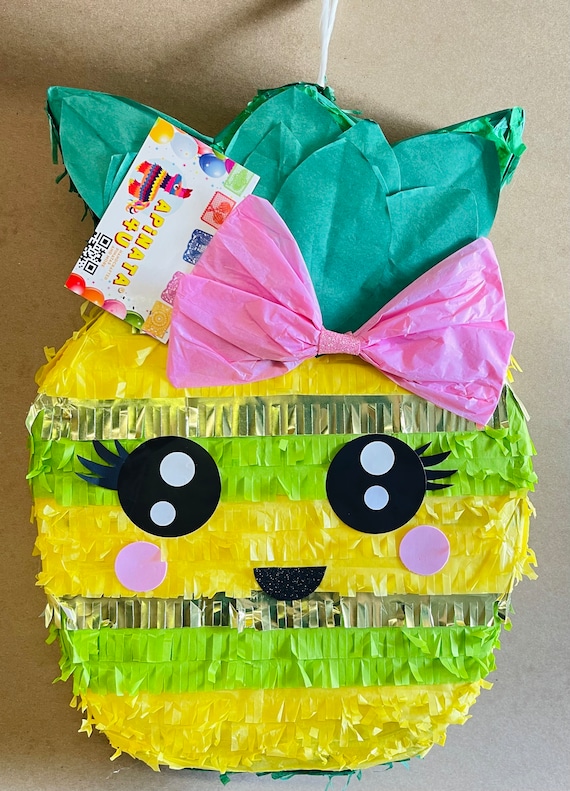This photograph captures a charming, cartoon-style piñata designed to resemble a pineapple, set against a light brown mottled background. The body of the piñata features paper fringes arranged in horizontal lines, alternating in colors: a base yellow line, followed by lime green, a small gold line, a thicker yellow line, another thick lime green line, a thin gold stripe, and another thick yellow line, which is partly obscured by various elements. At the top of the piñata, there are dark green, stylized paper leaves emanating behind a bright pink paper bow, enhancing its playful design. The piñata’s face is adorned with large, round black eyes, each with two white reflective circles and four pointed black eyelashes on either side. There are pink circles beneath each eye symbolizing rosy cheeks and a cute black semicircle dotted with white, representing a smile. This piñata is tagged with a white label, which is illustrated with balloons, a llama piñata, and a QR code. The tag reads, “A piñata for U” in yellow text, highlighting its child-friendly nature. Additionally, a white string is attached at the top, indicating where the piñata can be hung.